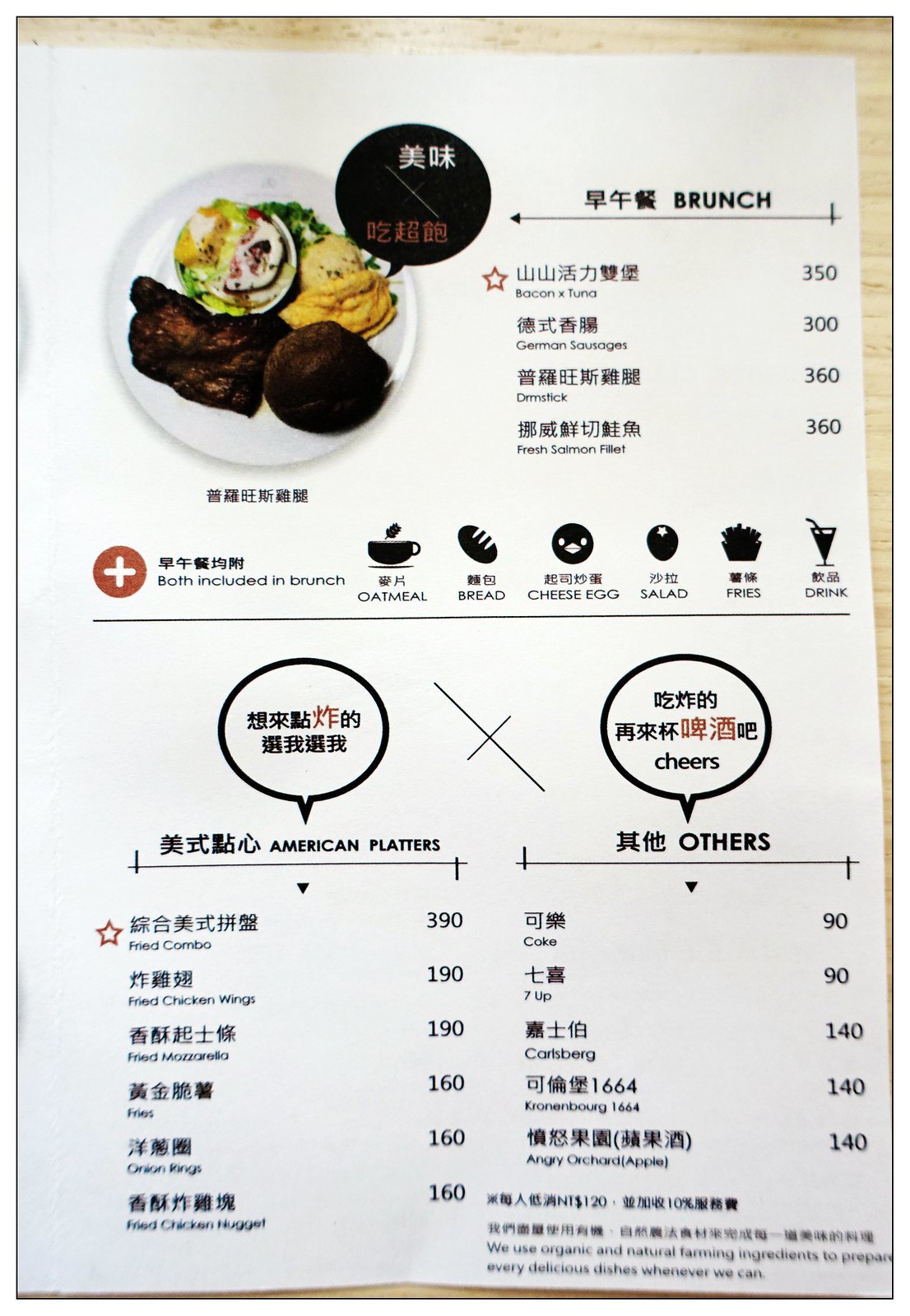A close-up image of a page from a Korean menu, featuring both Korean characters and English translations. The menu is structured with Korean text primarily to the left or above the English text, depending on the section.

At the top left of the image, there is a plate of food consisting of steak, potatoes, salad, and possibly mashed potatoes. To the right of this image, Korean characters are followed by the English heading "BRUNCH" in capital letters. Below this, the menu lists items with their corresponding prices: "Bacon and Tuna - 350," "Korean Sausage - 300," "Drumsticks - 360," and "French Salmon Fillet - 360." This section shows the Korean text above their respective English translations.

In the center of the image, there is a row of five icons representing various foods with Korean text below each icon. The icons, from center to right, depict "Omelet," "Bread," "Cheese Egg," "Salad," "Fries," and "Drink," and there is a note to the left indicating these items are included in the "BRUNCH."

The lower half of the menu is divided into two columns. The left column is labeled "American Platters," with items listed along with their prices: "Fried Combo - 390," "Fried Chicken Wings - 190," "Fried Mozzarella - 190," "Fries - 160," "Onion Rings - 160," and "Fried Chicken Nuggets - 160." 

The right column has a heading "Others" and includes beverages: "Coke - 90," "7 Up - 90," "Glassberg (or perhaps Charlesburg) - 140," and "Angry Orchard Apple - 140."